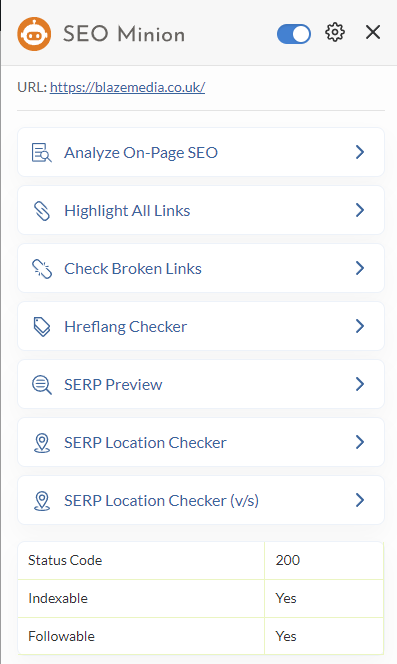This is a detailed screenshot captured in portrait mode, predominantly featuring a white background with a dark gray strip running across the top. In the upper left-hand corner, there's an icon depicting a space-themed figure enclosed within an orange circle, accompanied by the text "SEO Minion." The upper right-hand corner displays an active toggle button, a settings icon, and a black "X" for closing the interface.

Directly below this top section is a row showcasing a URL, "blazemedia.co.uk," underscored by a gray line. The main content area consists of seven sequentially arranged rows, each appearing to be live links, identifiable by their blue arrow indicators at the end and small icons to their left.

The seven links are labeled as follows:
1. Analyze On-Page SEO
2. Highlight All Links
3. Check Broken Links
4. Hreflang Checker
5. SERP Preview
6. SERP Location Checker
7. SERP Location Checker V/S

Beneath these links, a chart is visible. The left side of the chart is labeled with "Status Code," "Indexable," and "Followable." Correspondingly, the right side lists the status code as "200," with both "Indexable" and "Followable" marked as "Yes." 

This intricate screenshot appears to be from SEO Minion, offering an array of tools and statuses for analyzing web pages and their SEO metrics.